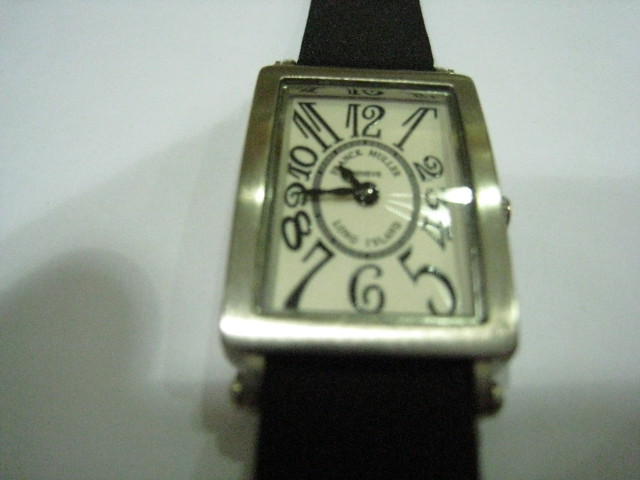The image depicts a uniquely designed wristwatch with a rectangular face. The watch features numbers in a whimsical, elongated style ranging from 1 to 12. The center of the watch face contains a small, black oval that appears to bear an inscription, potentially reading "something Miller" or "France Miller," though the exact wording is unclear. The watch frame is made of a lustrous silver metal, adding a touch of elegance to the quirky design. The watch is affixed to black straps, providing a classic contrast to the shininess of the frame. The entire watch is set against a white background, which is not fully discernible, and a shadow is visible at the bottom part of the image, giving depth to the scene.